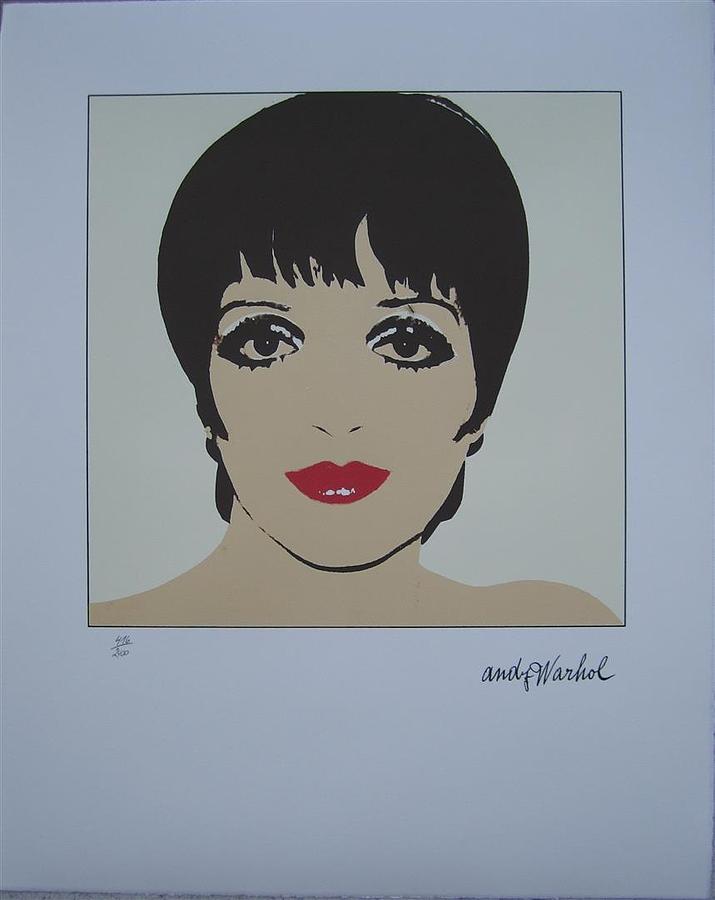This is a photograph capturing an iconic portrait of Liza Minnelli by Andy Warhol. The artwork is a limited edition print, numbered 416 out of 2400, showcasing Warhol's distinctive style. The composition is housed within a vertical rectangle featuring a periwinkle blue background, with the actual print itself being square and situated towards the upper part of the rectangle. This close-up of Minnelli prominently displays her face and bare shoulders against a light-colored backdrop. Her short, dark bob frames her face, with shaggy bangs nearly touching her eyebrows. Minnelli's signature dark eyes and bright red lipstick are vividly portrayed, alongside slight highlights above her eyelids and on the interior parts of her eyes. Her skin is rendered in a natural flesh tone, and her gaze is direct. A subtle, narrow shadow under her chin adds depth. Warhol’s name is inscribed in script on the bottom right, and the fractional number is on the bottom left, authenticating the piece. The print captures Minnelli's distinctive features with a minimalist yet striking approach, embodying a blend of boldness and subtlety typical of Warhol's work.